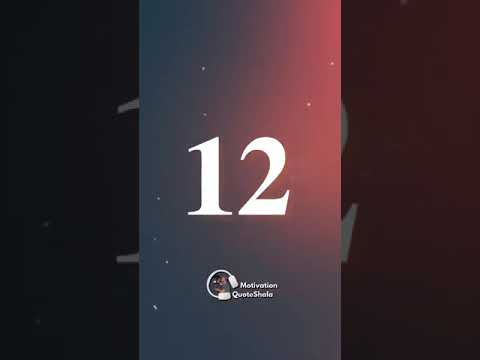The image is akin to a poster, divided into three vertical columns: the left and right columns are black, while the middle column transitions from gray on the left to red on the right, creating an infused blend. Central to the middle column, there's a prominent white number "12," the largest font in the image. Below it, a pair of white over-the-ear headphones is depicted, and next to the headphones, the words "Motivation Code Sala" or similar are written. The middle column's background also contains a larger, semi-transparent gray number "12," giving a layered effect. Scattered throughout this gray-red background blend are approximately eight white dots, resembling stars, which add a night sky-like ambiance to the image. The far left and right portions of the number "12" are subtly visible in the background, enhancing the layered, almost mirrored look.